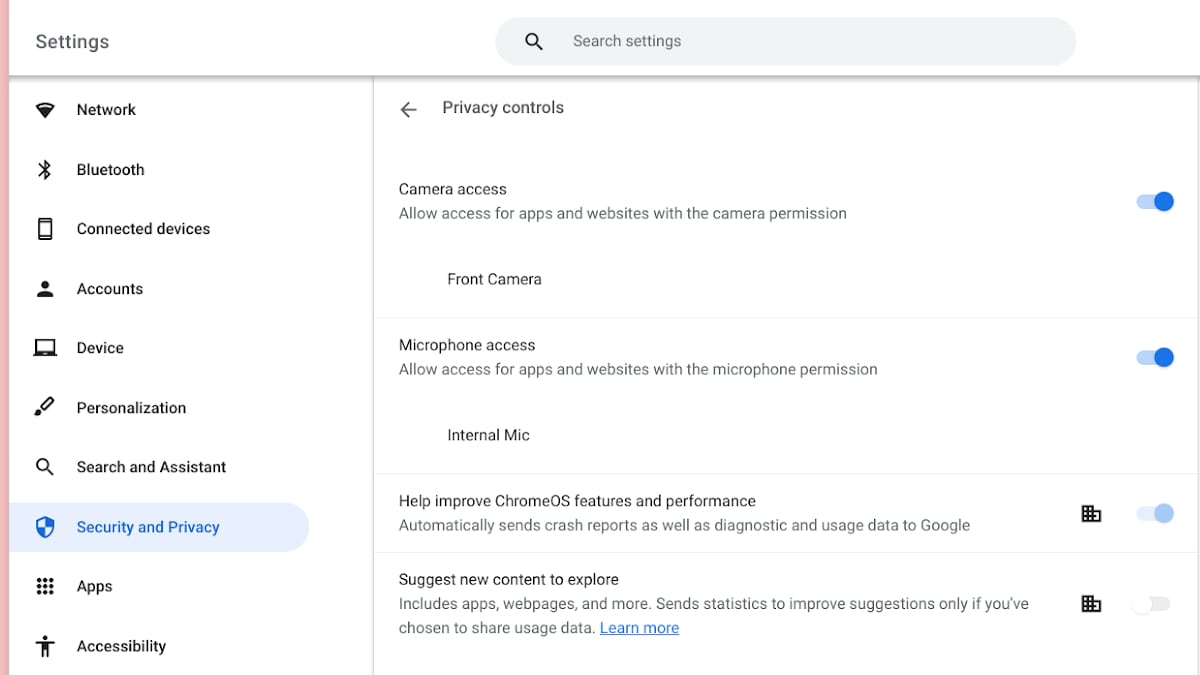A detailed and cleaned-up caption for the described image:

This image captures a screenshot from a computer or possibly a wide-screen mobile device, displaying the "Settings" menu in a graphical user interface. At the top of the screen, the word "Settings" is displayed prominently in black font. Just below it, in a gray bar, there is a search field labeled "Search settings" accompanied by a magnifying glass icon.

Along the left side of the screen, there is a vertical list of icons and corresponding labels, each representing different sections within the settings menu. The icons and their labels are as follows:
1. A connectivity icon labeled "Network."
2. An icon resembling a bee labeled "Bluetooth."
3. An icon depicting a cell phone labeled "Connected devices."
4. A silhouette of a person labeled "Accounts."
5. An icon of a computer labeled "Device."
6. A pen icon labeled "Personalization."
7. A magnifying glass icon labeled "Search and assistant."
8. A shield icon labeled "Security and privacy," which is highlighted, indicating it has been selected.
9. An icon labeled "Apps."
10. A stick figure icon labeled "Accessibility."

This organized layout provides a user-friendly interface for navigating through various system settings.